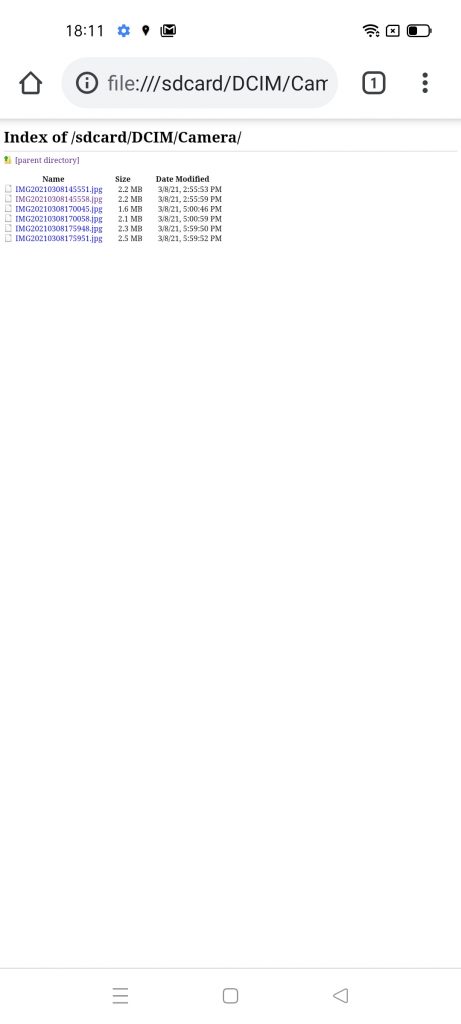A close-up image of a cell phone screen showing a simple, text-dominant interface devoid of artistic elements. The interface features no photos, drawings, or elaborate designs. In the top left corner, there are icons for "Settings" gear, a location pin, and an envelope symbol, alongside the time display "18:11". The top right corner indicates the wireless connection status and a battery icon displaying a 40% charge. Below these icons, an address bar shows the path: "file:///sdcard/DCIM/CAM...", which is truncated. Beneath this, the text reads "Index of /sdcard/DCIM/camera/" followed by the option "Parent Directory."

The main section is divided into three columns labeled "Name," "Size," and "Date Modified." Each column lists six items. The first item under "Name" is "IMG_2021-0308145551.jpg," with a "Size" of "2.2 MB" and a "Date Modified" timestamp of "3/8/21 2:55:53 PM." Similar entries populate the remaining rows, delivering consistent information across all six listings.